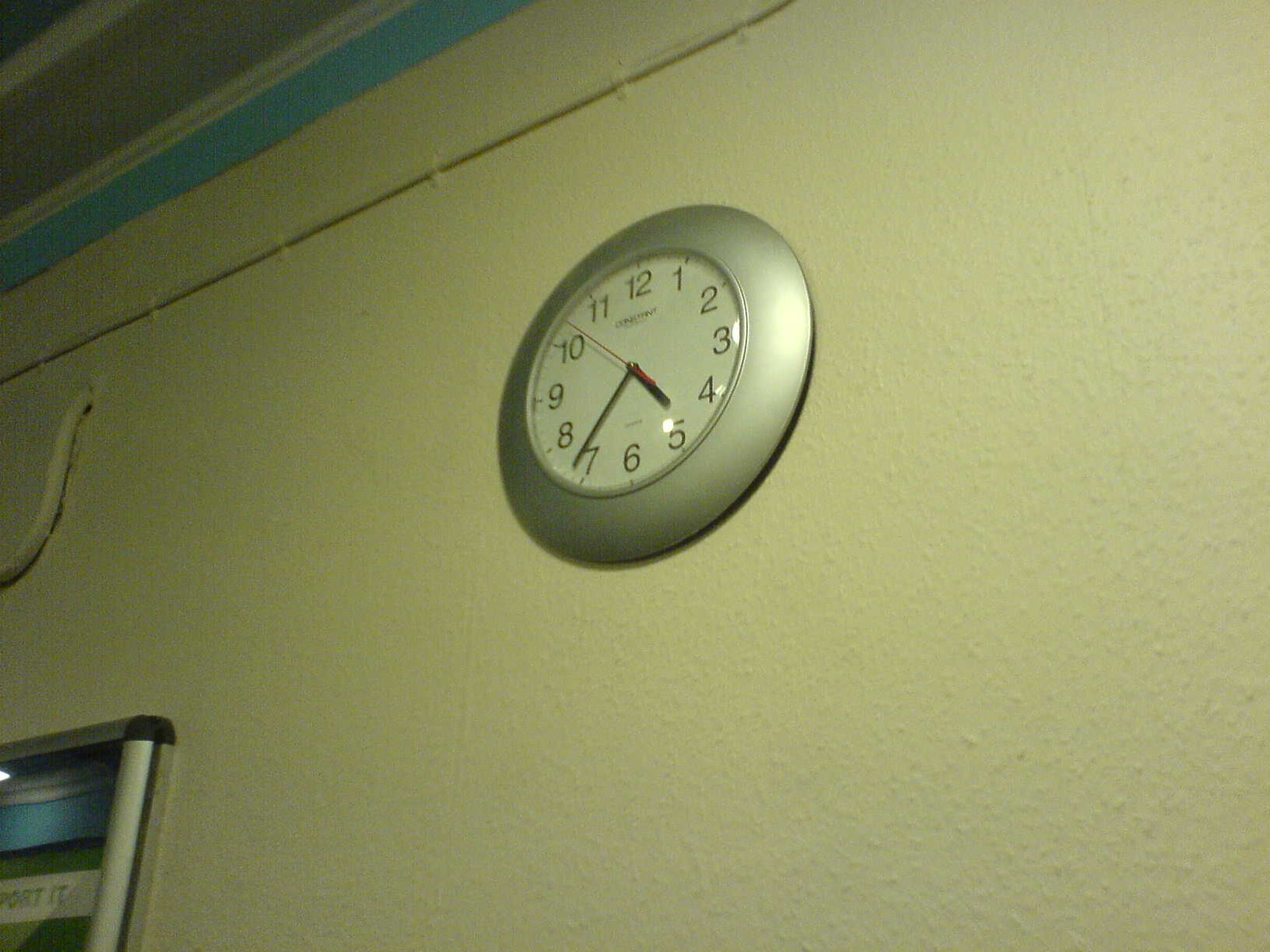This gritty, older photograph captures a silver round clock mounted on an off-white, textured, popcorn-style plaster wall. The clock, illuminated by artificial light in a dimly lit room, casts a faint shadow on the wall. The clock face is white with black numerals from 1 to 12, and it features three hands—black hour and minute hands, and a red second hand. Above the clock extends a thin, industrial pipe-like object. The lower part of the image reveals a silver object accented with green, white, and blue colors, and the room’s ceiling shows a teal rim and gray molding. Additionally, there's a framed sign to the bottom left of the clock, suggesting an indoor, possibly basement setting devoid of natural light. The time displayed on the clock reads 4:36, indicating it is likely early morning due to the room’s darkness.